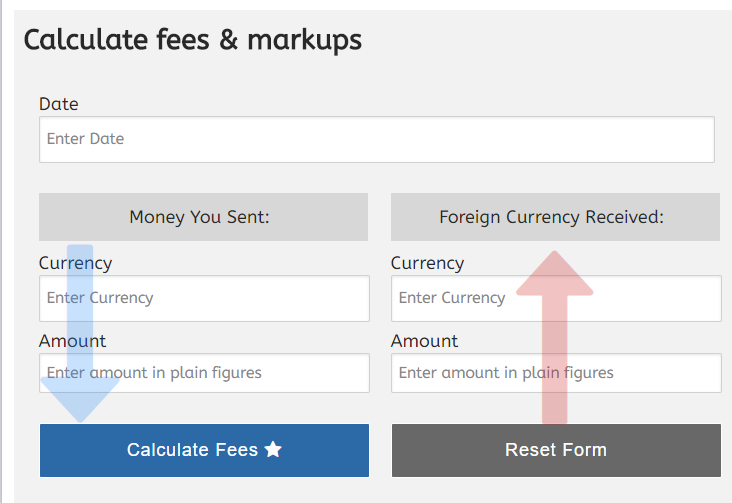The image showcases a "Calculate Fees and Markups" screen with a grayish background. In the top left corner, it prominently displays the title "Calculate Fees and Markups." Below the title, there's a labeled bar with the text "Enter Date." The interface is split into two main sections, each with a distinctive heading: "Money You Sent" on the left and "Foreign Currency Received" on the right.

Under the "Money You Sent" section, there is a subheading labeled "Currency" followed by an input bar that prompts the user to "Enter Currency here." Below this, there's another subheading labeled "Amount" with a corresponding input bar for entering the amount in plain figures. A notable element in this section is a blue button labeled "Calculate Fees," adorned with a star icon. A blue arrow points downward from the "Money You Sent" section to this "Calculate Fees" button.

In the "Foreign Currency Received" section, a similar layout is followed. It starts with a "Currency" subheading and an input bar that says "Enter Currency." Below that, there's an "Amount" subheading accompanied by a bar for entering the amount in plain figures. At the bottom of this section, there's a dark gray button labeled "Reset Form." A red arrow points upwards from this "Reset Form" button towards the "Foreign Currency Received" heading.

The rest of the image is white beneath these elements, providing no additional information below the two buttons. This clean and organized layout guides the user through entering relevant currency details and calculating associated fees and markups while offering the option to reset the form if necessary.